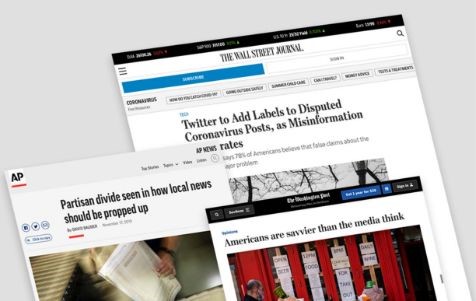This image is a horizontally oriented screenshot with a light gray background, featuring a layered arrangement of three illustrated newspaper pages at a left-leaning angle. The background page, partially visible at the top, is labeled "The Wall Street Journal" with a black banner. Its headline reads, "Twitter to Add Labels to Disputed Coronavirus Posts as Misinformation," followed by a subheading titled "Rates." A partial black and white photograph of trees is faintly visible at the top of this page.

Laid over the background page, the upper left paper is identified as an AP publication. Its prominent headline reads, "Partisan Divide Seen in How Local News Should be Propped Up." Beneath this, another photograph depicts a man holding a newspaper, although the bottom edge is cut off.

Overlapping both the background and the leftmost page, the smallest newspaper on the top right features the headline, "Americans are Savvier than the Media Think." Below this headline, a photograph showcases red banners with white pages mounted on wooden beams, with a man positioned in the lower-left corner. Both the background and the rightmost newspaper pages are topped with a horizontal black border.